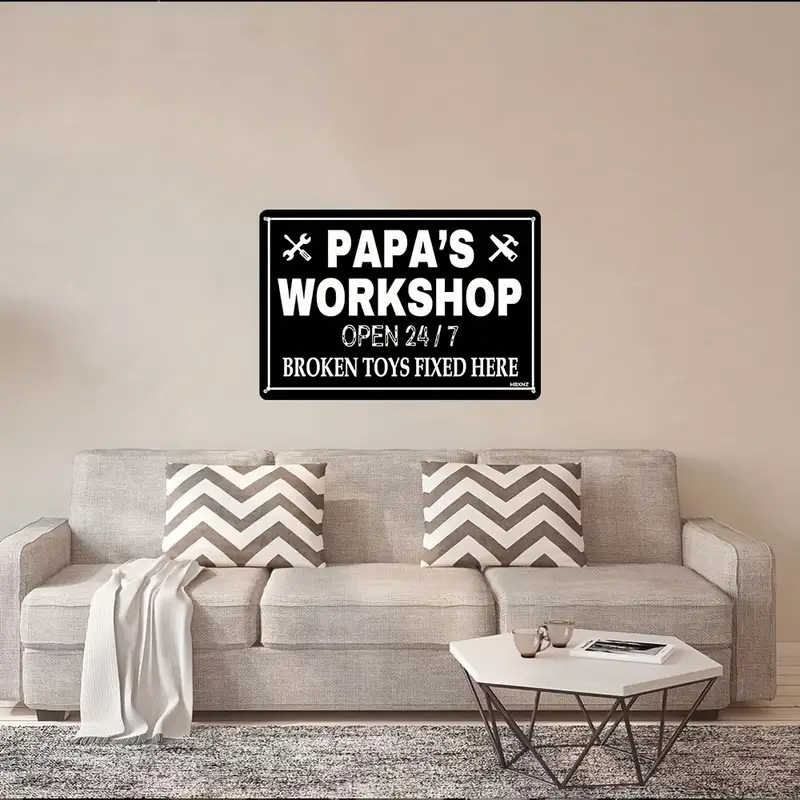This indoor photograph features a meticulously staged living room scene. Dominating the center is a light gray, three-seat couch with armrests and cushions that match the sofa's fabric. Accenting the couch are two throw pillows adorned with a chevron pattern of yellow and gray diagonal stripes, contrasting with the gray blanket draped over the left side of the couch. The floor showcases light-colored wooden slats, topped with a speckled gray area rug. To the right of the couch is a hexagon-shaped coffee table bearing two glass teacups and a coffee table book. Central to the composition, hanging on a faint brown wall with a peachy undertone, is a black rectangular sign. The sign reads in white text, "Papa's Workshop, open 24-7, broken toys fixed here," flanked by a white silhouette of a wrench and screwdriver on the left and a hammer and saw on the right.